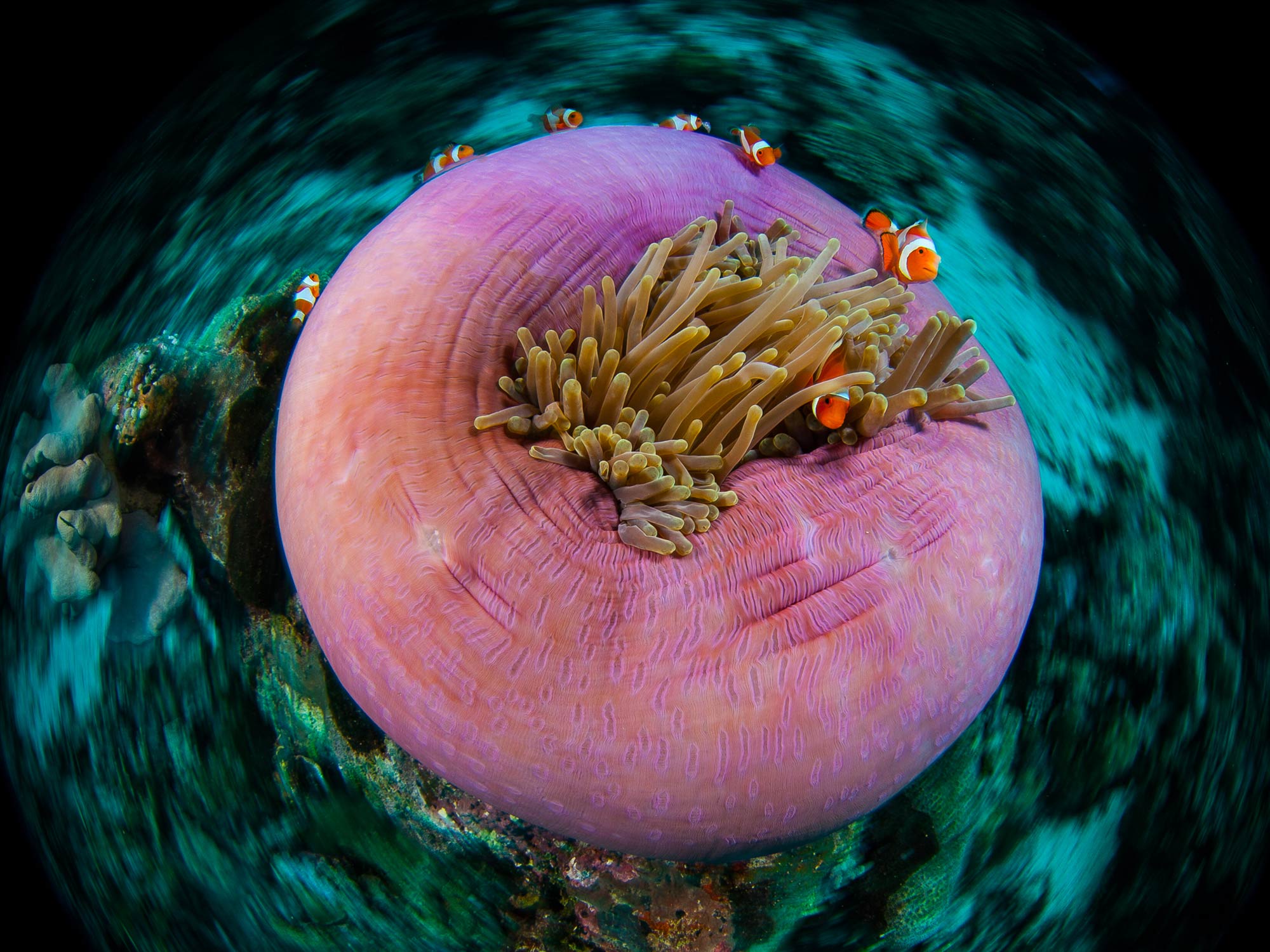In this underwater photograph, a mesmerizing pink and purple anemone with yellow-tipped tentacles anchors the scene. Nestled amidst a swirling backdrop of deep blues, teals, and grays, this vibrant marine life feature captures the eye. Darting around the anemone are several tiny clownfish—reminiscent of those from the movie "Finding Nemo"—with seven clearly visible. One clownfish is tucked within the tentacles, while others swim energetically around, possibly seeking refuge in the anemone's inviting shelter. The seafloor beneath, though out of focus, reveals hints of coral and scattered rocks, adding to the enchanting oceanic ambiance.